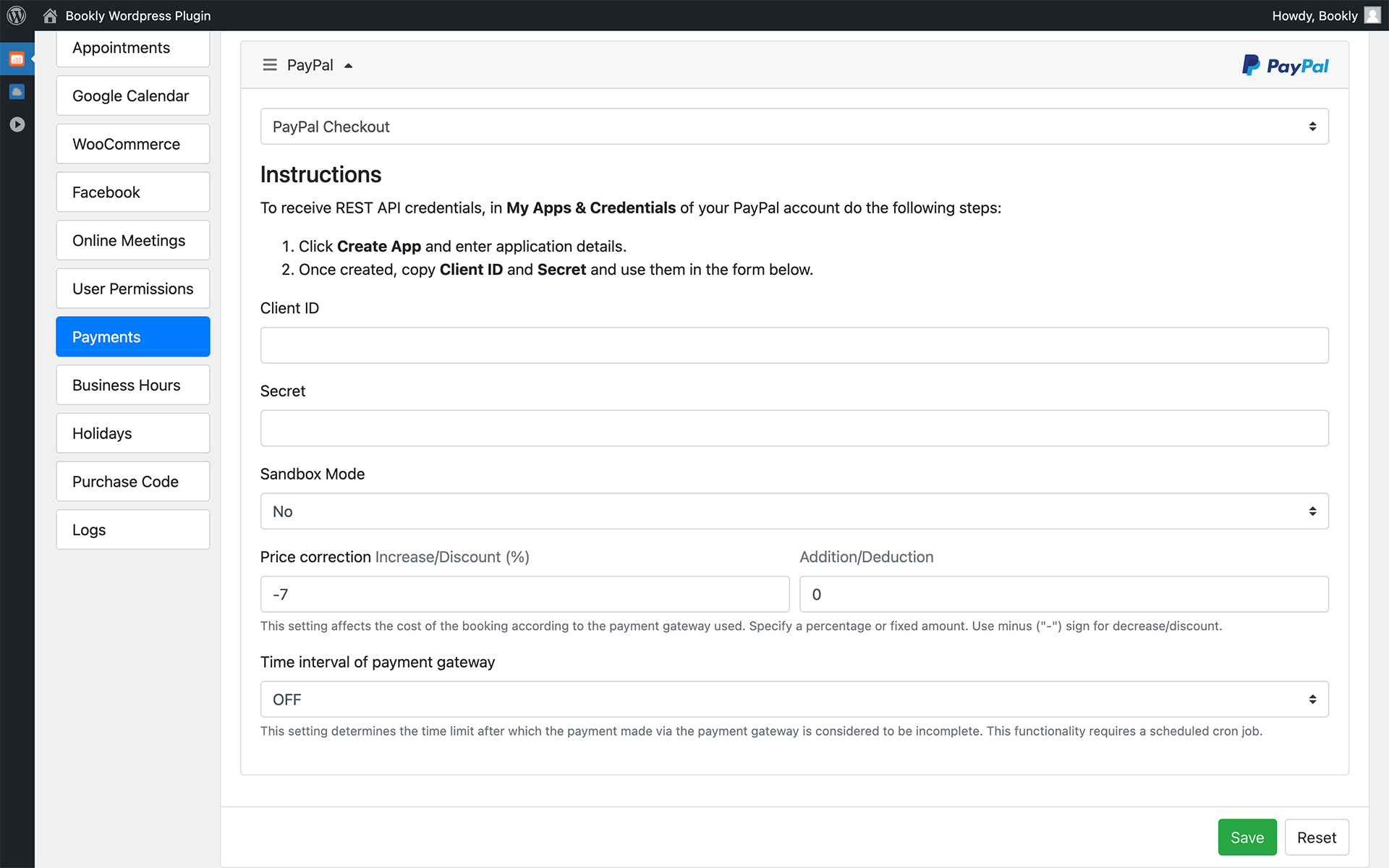**Detailed Caption:**

The image is a screenshot of the WordPress dashboard, specifically within the settings of the Bookly plugin, focusing on the payments section. 

**Layout and Interface:**
- **Top Bar:** At the top, the header includes the plugin's name and a user greeting "Howdy Bookly" situated on the right side.
- **Sidebar:** On the far left, a gray sidebar features icons for various menu options. These options include:
  - **Appointments**
  - **Google Calendar**
  - **WooCommerce**
  - **Facebook**
  - **Online Meetings**
  - **User Permissions**
  - **Payments** (highlighted in blue with white text)
  - **Business Hours**
  - **Holidays**
  - **Purchase Code**
  - **Logs**

**Main Content Area:**
- The larger main column is dedicated to the settings for the payment gateway, currently set to PayPal. Key elements in this area are:
  - **Title and Logo:** At the top left, it shows "PayPal" alongside the PayPal logo.
  - **Drop-down Menu:** Below that, there's a drop-down menu displaying "PayPal checkout" as the selected option.
  - **Instructions Section:** A section with a white background and black text provides detailed instructions for configuring REST API credentials from the PayPal account. The steps include:
    1. Click "Create" and enter application details.
    2. Once created, copy the "Client ID" and "Secret" and input them into the form below.
  - **Form Fields:** The form includes the following input fields:
    - **Client ID**
    - **Secret**
    - **Sandbox Mode:** A drop-down list with "No" selected.
    - **Price Correction:** A field labeled with "Increase or Discount by percentage," showing a value of 7.
    - **Addition/Deduction:** A field with a value of 0. Accompanying text explains that this setting affects the booking cost according to the payment gateway used and allows a percentage or fixed amount, with a minus sign for discounts.
    - **Time Interval of Payment Gateway:** Set to "Off," with a description stating that this setting determines the time limit after which an incomplete payment is recognized. It notes that a scheduled cron job is required for this functionality.
- **Action Buttons:** At the bottom right corner, there are two buttons:
  - **Save:** Green with white text.
  - **Reset:** White with black text.